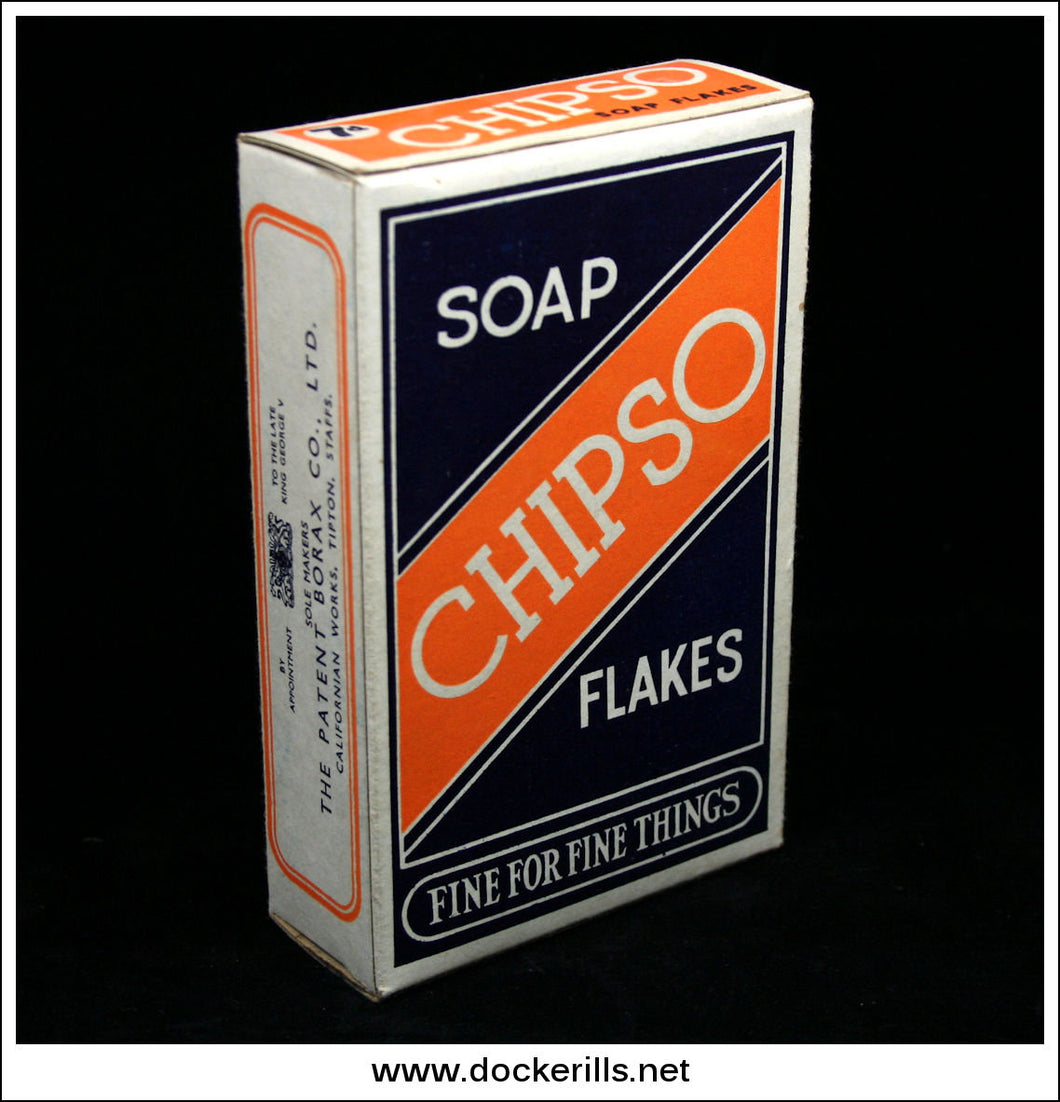The image features a vintage box of soap flakes prominently displaying the brand name "Chipso" with a distinctly old-fashioned design. The box predominantly sports an orange, white, and black color scheme with an orange banner across the middle that reads "Chipso" in white letters. The name "SOAP" appears above the banner, while "FLAKES" is written below it, both in white text against a blue background that forms the top and bottom triangles of the box's front. The slogan "FINE FOR FINE THINGS" is positioned at the bottom of the box in white font. The side of the box is visible, showing the text "THE PATENT BORAX COMPANY LIMITED CALIFORNIAN WORKS SOAP MAKERS." On the top, it repeats "CHIPSO" with an orange background and indicates it was priced at "SEVEN CENTS." The entire box is set against an opaque black background, and a website link, "www.dockerills.net," is visible at the bottom edge of the image.